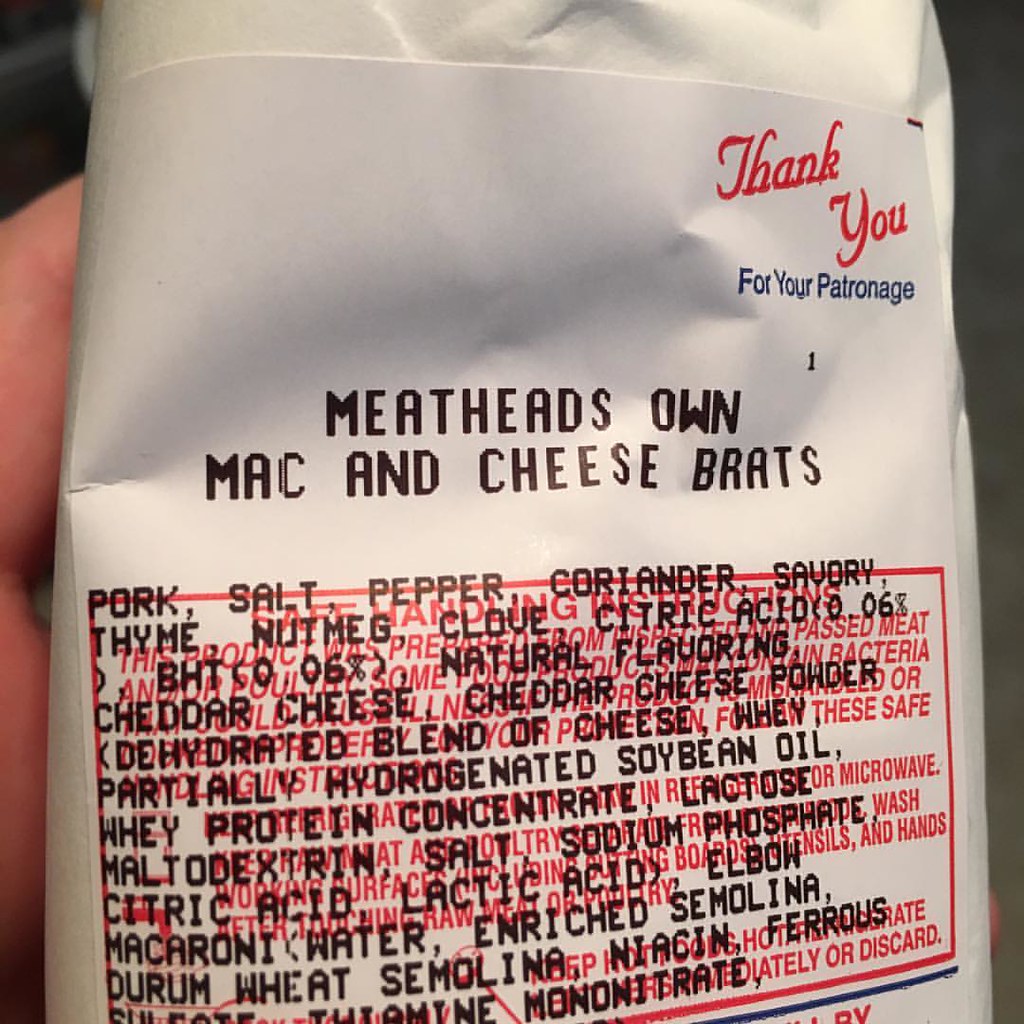In this close-up photograph, a hand holds a neatly wrapped package of white butcher paper, secured with a large white label that dominates the frame. The index finger and a portion of the hand are visible in the upper left corner, emphasizing the personal touch. The top right corner of the label reads, "Thank you for your patronage" in elegant, small text. Central to the label, bold text proudly announces the product as "Meatheads Own Mac and Cheese Brats." Below this, a red rectangle is meant to display the safe handling instructions. However, the instructions are partially obscured by additional text listing the ingredients of the brats, making the safety information difficult to decipher. The overall effect combines the homely charm of butcher-wrapped goods with a touch of homemade craftsmanship.